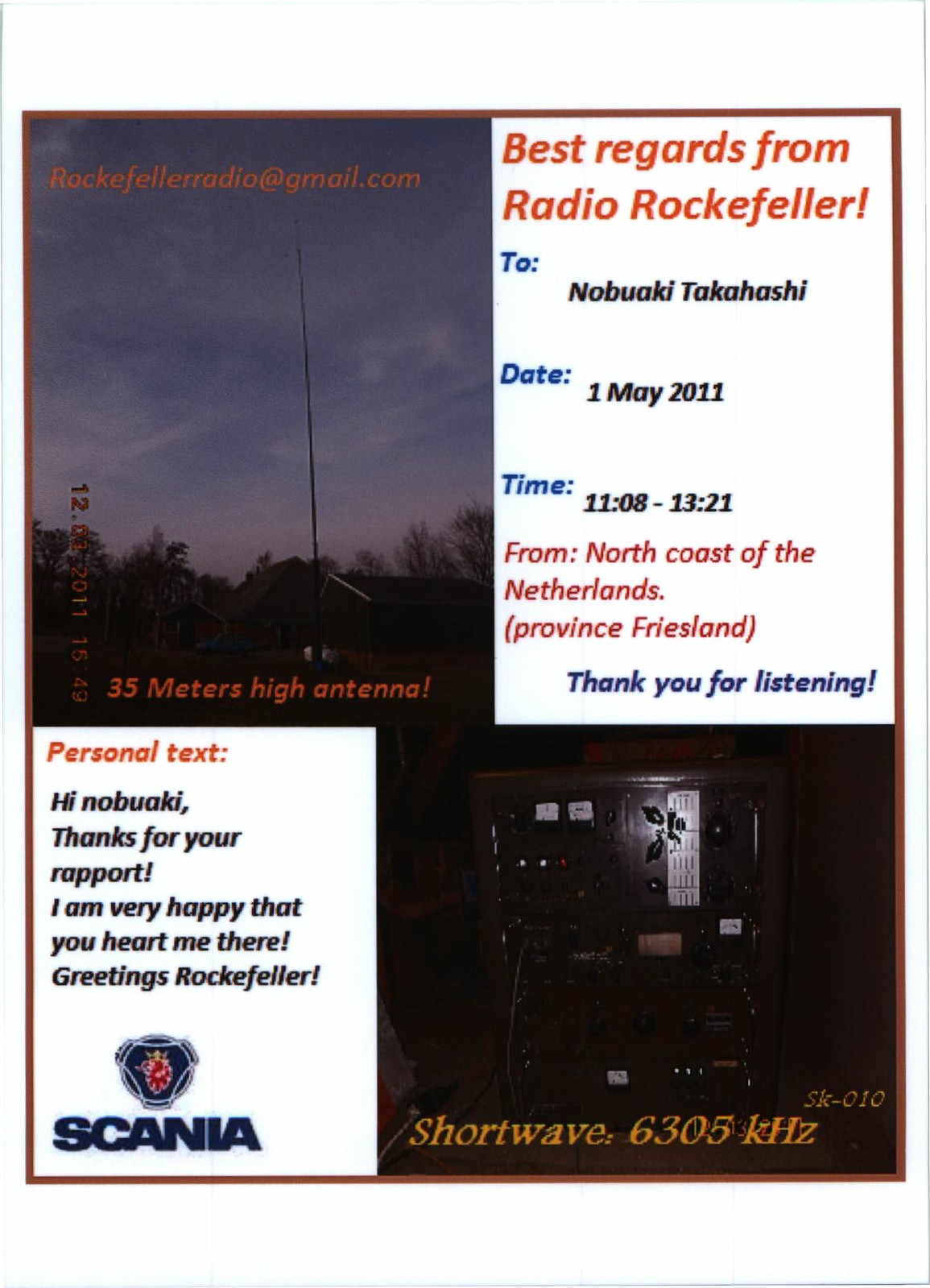The image serves as a computer-generated thank-you note set against a photograph of an outdoor scene featuring a dark sky and the rooftops of some houses. Dominating the upper left corner is an antenna labeled with orange text stating "Rockefeller Radio at gmail.com" and "35 meters high antenna, shortwave 6305 KHZ." In the top right, an overlaid white box contains a message in orange and blue text: "Best regards from Radio Rockefeller to Nobuo Aki Takahashi, Date: 1st May 2011, Time: 1108 to 1321, From the North Coast of the Netherlands, Province: Friesland. Thank you for listening." Another similar white box appears in the bottom left corner with a personalized note: "Hi Nobuo Aki, thanks for your report. I am very happy that you heard me there. Greetings, Rockefeller." The lower left corner also features a blue and red logo, which includes a lion's head with a crown encircled by a ring, alongside the text "SCANIA."